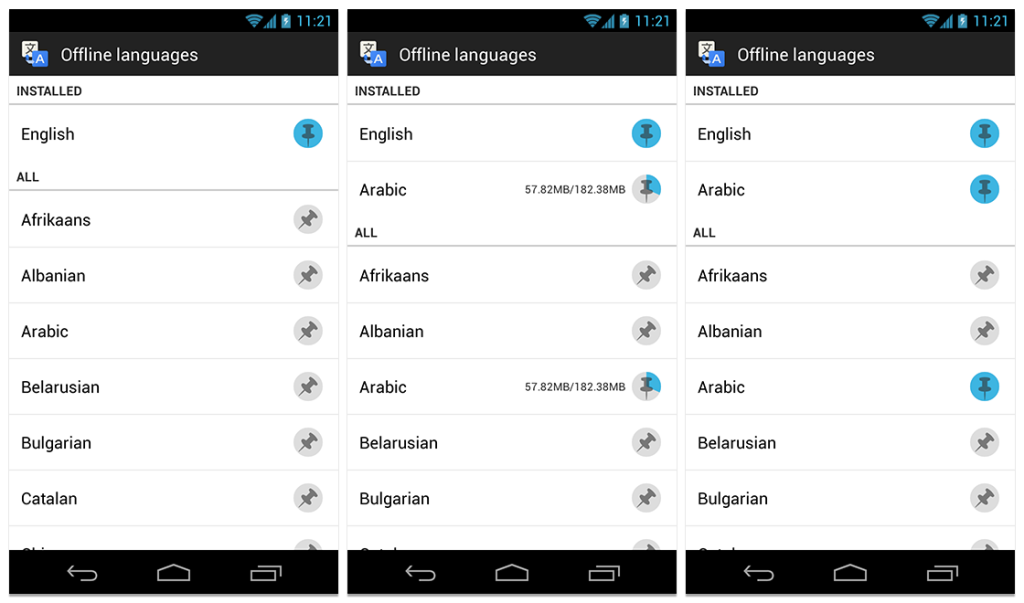The image consists of three sequential phone screenshots, all captured at the same time (11:21) as indicated by the clock on the top right corner of each image. The battery icon shows it is fully charged and still connected to a charger. Each screenshot displays a section from a phone's "Offline Languages" settings.

1. **First Screenshot (left):** The background of the interface is black. The screenshot shows a list titled "Installed Languages" starting with English, marked as installed. Below this, languages appear in alphabetical order: Afghan, Albanian, Arabic, among others.
   
2. **Second Screenshot (middle):** Similar to the first, this screenshot shows English as an installed language. Arabic is in the process of being downloaded, which is evident from a progress bar. Beneath these, additional available languages are listed.

3. **Third Screenshot (right):** English and Arabic are both marked as fully installed. Below these installed languages, the list continues with other available languages.

This sequence demonstrates the progression of downloading and installing the Arabic language alongside previously installed English, within the phone’s language settings.